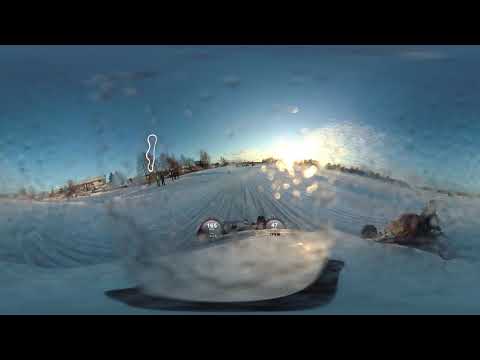The image depicts a winter scene viewed through a wet, raindrop-covered windshield or piece of glass, creating a distorted effect. The foreground features an unidentifiable object resembling a sled or boat with two circular items marked with the numbers "146" and "47." These objects appear to be going down a snowy hill, as evidenced by the sled marks or tracks veering in various directions. The ground is covered in snow with blue tints, and the sky is a clear, vibrant blue without any clouds, indicating a sunny day. In the middle left of the background, there are sparse trees and a few small, indistinct figures, possibly people, standing around. Farther in the distance, there are faint outlines of houses, barely discernible from this distance. The entire scene has a glary area that reflects off the raindrops, adding to the overall blurriness and making it difficult to ascertain specific details clearly.